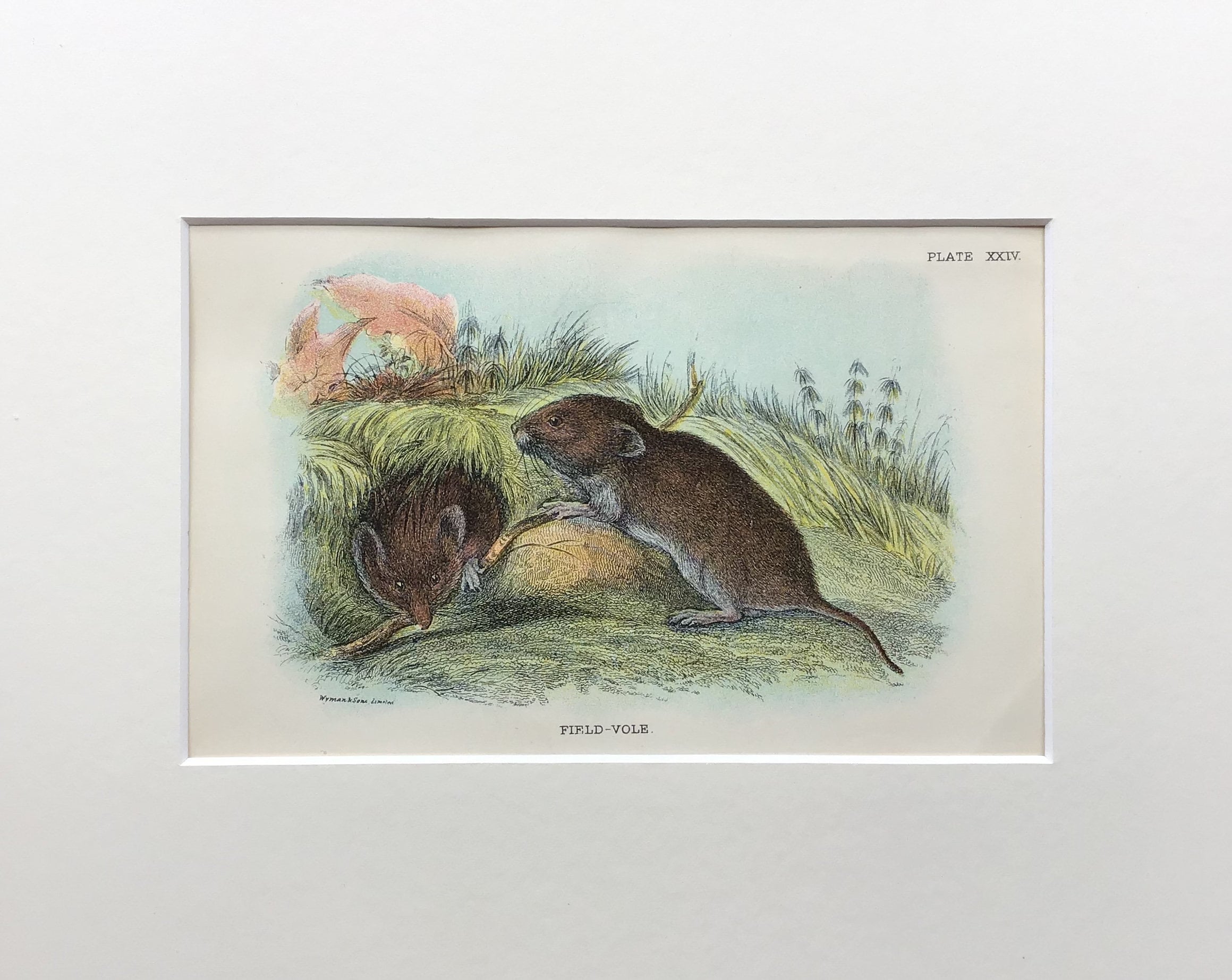This painting, titled "Field Vole," is a detailed depiction of a natural scene presented on a white background with a thick white mat border. Centered in the artwork, two brown field voles, which resemble mice, are portrayed amidst a setting of green and brown grasses. One vole is facing the viewer, displaying both eyes and one paw, while the second vole is shown in profile with only one eye visible, and both a front and back paw near its tail. The voles, with their small, white feet, appear almost endearing.

Surrounding the voles, the grass appears as a collection of sketched lines, mingled with twigs and a few reddish-orange leaves located in the top left corner of the painting. A light pink leaf is also seen in the same vicinity, adding contrast to the scene. The sky in the background is a muted, slightly bluish tone, enhancing the overall natural atmosphere.

At the top right corner, the painting is marked "Plate XXIV" in Roman numerals. The bottom middle of the piece is inscribed with the title "Field Vole" in black letters, though the precise spelling varies slightly across descriptions. Additionally, the artist’s signature appears at the bottom left, although it is not legible without closer inspection.